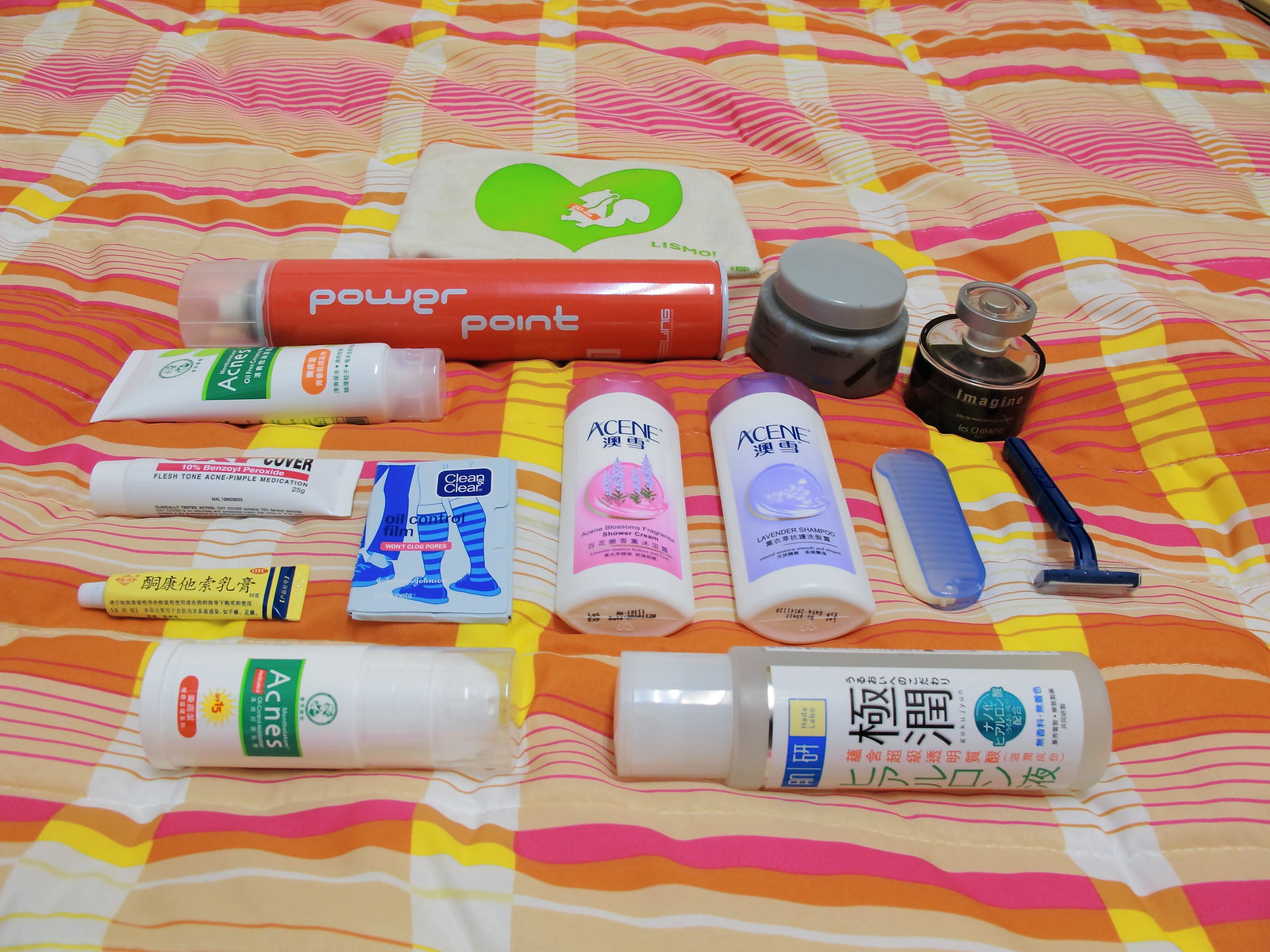Several beauty products are meticulously arranged on a vibrant striped comforter, composed of white, pink, dark orange, light orange, and yellow hues. At the bottom center of the image are two bottles placed cap-to-cap. The left bottle is white with a green label that reads "Acnes," while the right one is a clear bottle with a white label adorned with some characters. Positioned behind the clear bottle is a blue disposable razor, adjacent to which is an unidentifiable purple object. Nearby, two similar bottles, one purple and one pink, are lined up next to a "Clean & Clear" packet. To the left of this setup, there's a small yellow tube with a white tube featuring pink lettering placed on top. 

Continuing upwards, there is another white bottle with a green label matching the design of the first bottle mentioned. Towering behind this cluster is a large orange hairspray bottle labeled "PowerPoint." At the very back of the arrangement, a small white makeup bag embellished with a green heart and a cute animal figure can be seen. To the right of the hairspray bottle sits a small black and gray pot accompanied by a petite spray bottle.

The entire ensemble is thoughtfully displayed, showcasing an array of skincare and beauty essentials against a colorful and eye-catching backdrop.